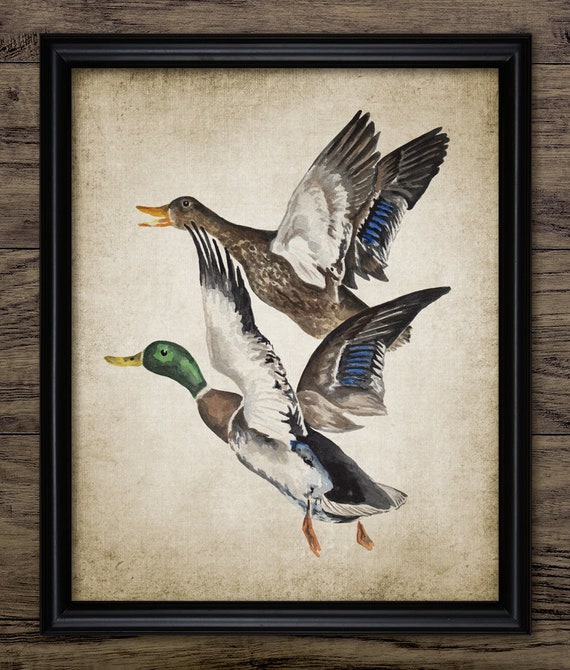This detailed painting is encased in a black frame and set against a brownish-gray, wood-slatted wall. The artwork features an off-white background with tan shading in each corner. At the bottom center of the image is a male mallard duck characterized by its distinctive green head and tan-and-white neck ring. The duck is in flight, heading from the bottom right to the top left, with its fully open wings displaying striking blue feathers near the base and dark tips. Its back is black, and its belly is white. Above the male, a mottled brown and white female mallard duck, identifiable by her yellow beak, is also in flight. Her wings are raised more directly over her back, revealing the white underside and the blue feathers near the base. Both ducks appear to be lifting off into the air together, evoking a sense of romantic companionship as they soar into the distance.